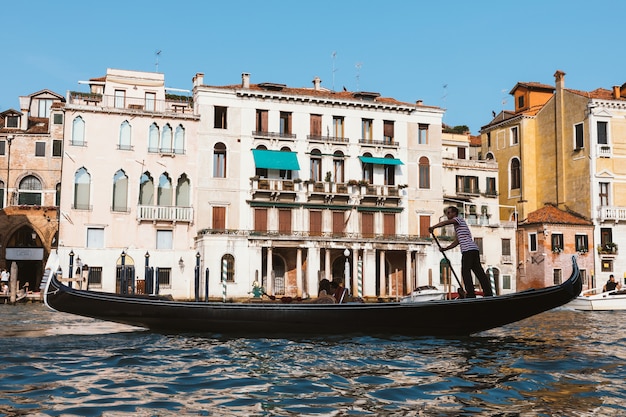This vibrant photo captures a quintessential Venetian scene on a sunny day, characterized by a bright blue sky. The focal point is a traditional gondola, sleek and black, with the signature curved ends distinctive to Venice. A gondolier, dressed in a red and white striped shirt and black pants, stands at the back, skillfully maneuvering the boat with a long paddle. Seated in the gondola are two passengers, though the details are blurred due to the image resolution. They glide along a canal with gently rippling water that reflects the azure of the sky.

The backdrop features an array of buildings, mostly four stories tall, showcasing classic Venetian architecture. The buildings boast a mix of beige, cream, and light terracotta hues. A particularly eye-catching structure has teal awnings and terracotta rooftops, juxtaposed against the other buildings with their numerous windows and a few smokestacks. Additionally, some windows are adorned with blue shades, providing a splash of color that stands out in the scene. Antennas dot the rooftops, emphasizing the urban landscape.

In the distance, other boats are moored along the shoreline, and people can be seen enjoying the serene ambiance of Venice. The combination of architectural beauty, lively waterways, and clear skies encapsulates the charm and elegance of this renowned Italian city.